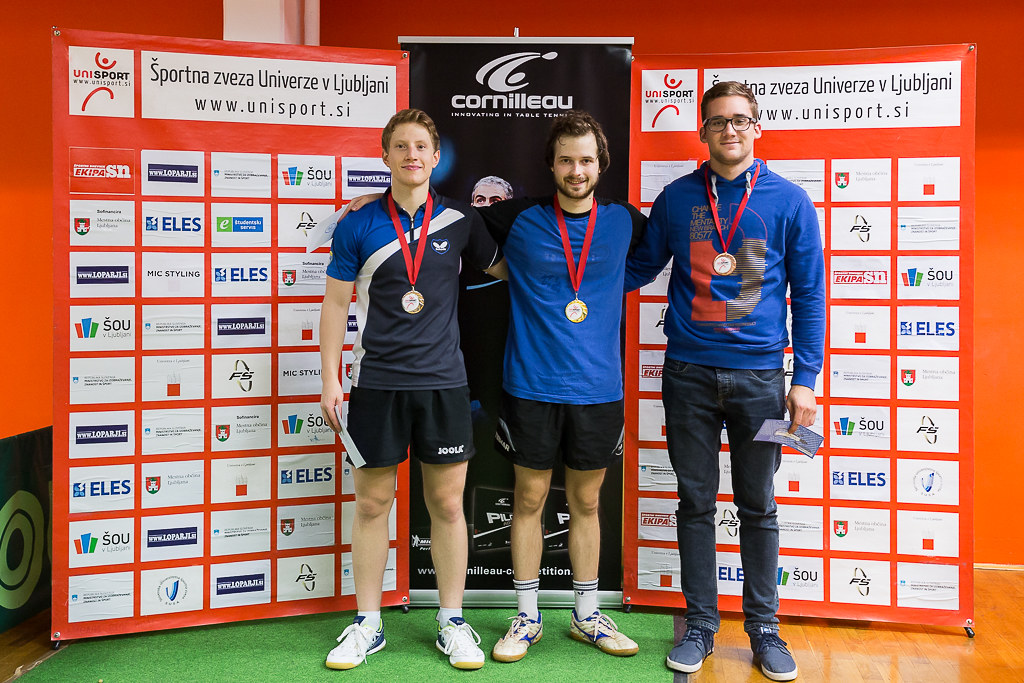The photograph captures three young Caucasian gentlemen standing in front of a sponsor-filled backdrop. The two on the left appear to be winners of a sporting event, wearing medals with red ribbons around their necks and dressed in athletic shorts and shirts. The gentleman on the right, possibly another athlete or their coach, is dressed in pants and is of similar age, adding an element of ambiguity to his precise role. The backdrop behind them features a grid of repeating sponsor logos, including one that prominently reads "Cornelio" and another related to "Unisport," both of which are set against a design that includes reddish-orange and black tones. The setting is modern with a combination of green astro-turf-like flooring on the left and hardwood flooring on the right, complementing the red walls visible behind the banners. The overall impression suggests a contemporary European sports event, promoting various sponsors with meticulous branding.